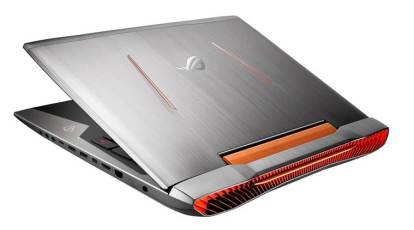The image depicts a high-end, metallic gray laptop on a white backdrop, partially open at roughly a 20-degree angle. The laptop's distinctive back design showcases orange ventilation ports and red elements, along with an orange hinge closure. The top lid, viewed from behind, features two orangish streaks and a logo. The base of the laptop, visible due to its open position, reveals a mix of black and gray keys on the keyboard. All the USB ports and other connections are situated on the right-hand side, visible on the left in the image.